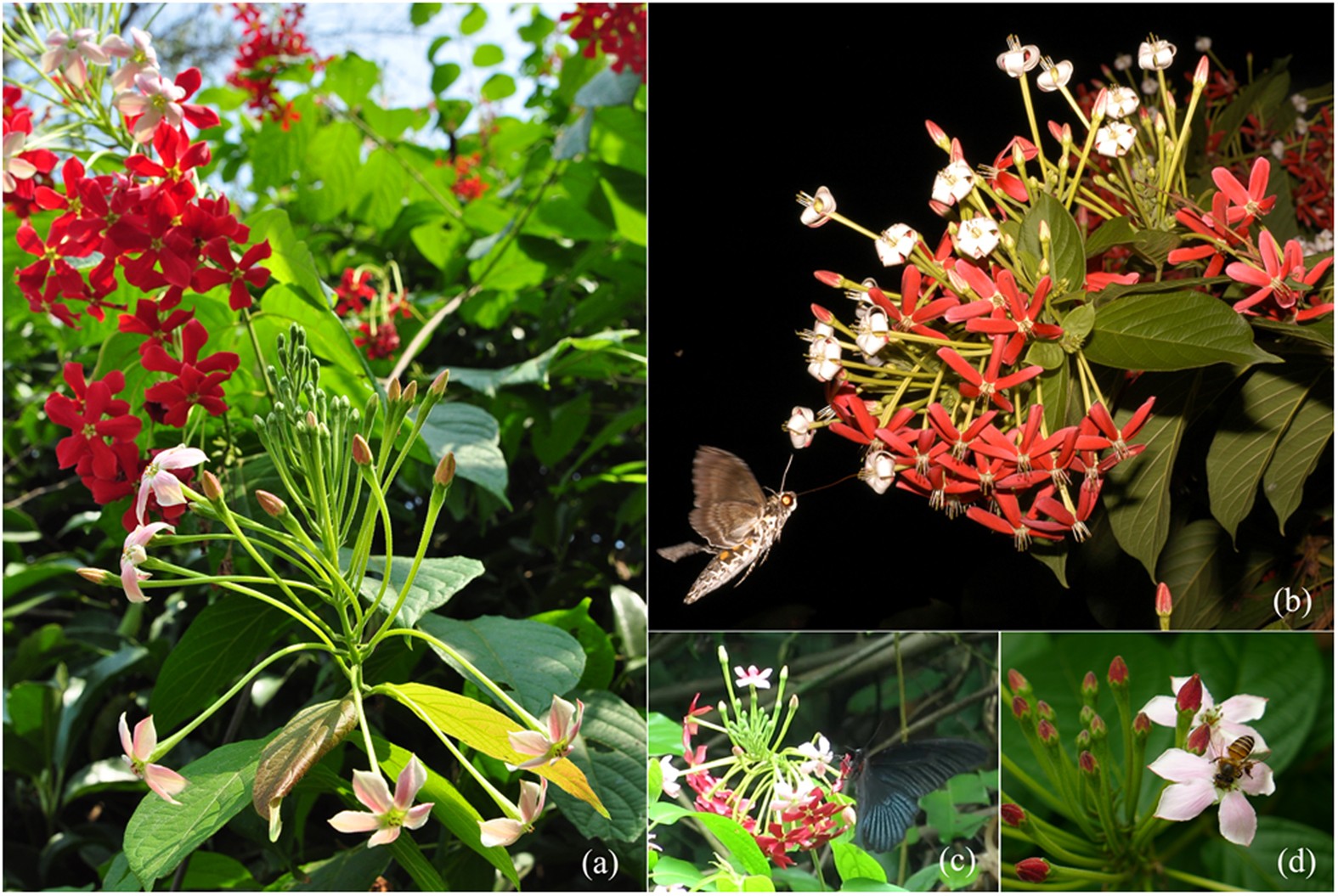The photograph collection showcases four distinct images labeled A, B, C, and D, providing a detailed study of two types of flowers in various arrangements. In image A, occupying the left half of the view, a striking red flower with five spread-out petals is prominently displayed alongside a lighter pink flower, whose petals bend backwards with a protruding center. Image B, filling the top three-fifths of the right side, continues the theme with similar flowers clustered together, and features a butterfly or moth in the bottom left corner. Image C mirrors the floral subjects, but with the red flowers angled downwards and the pink flowers aiming upwards. Finally, image D zooms in on the pink flower, highlighting its center with a bee perched delicately on it. The compilation captures the vibrant colors and intricate details of the flowers, accentuated by the contrast of their natural settings.